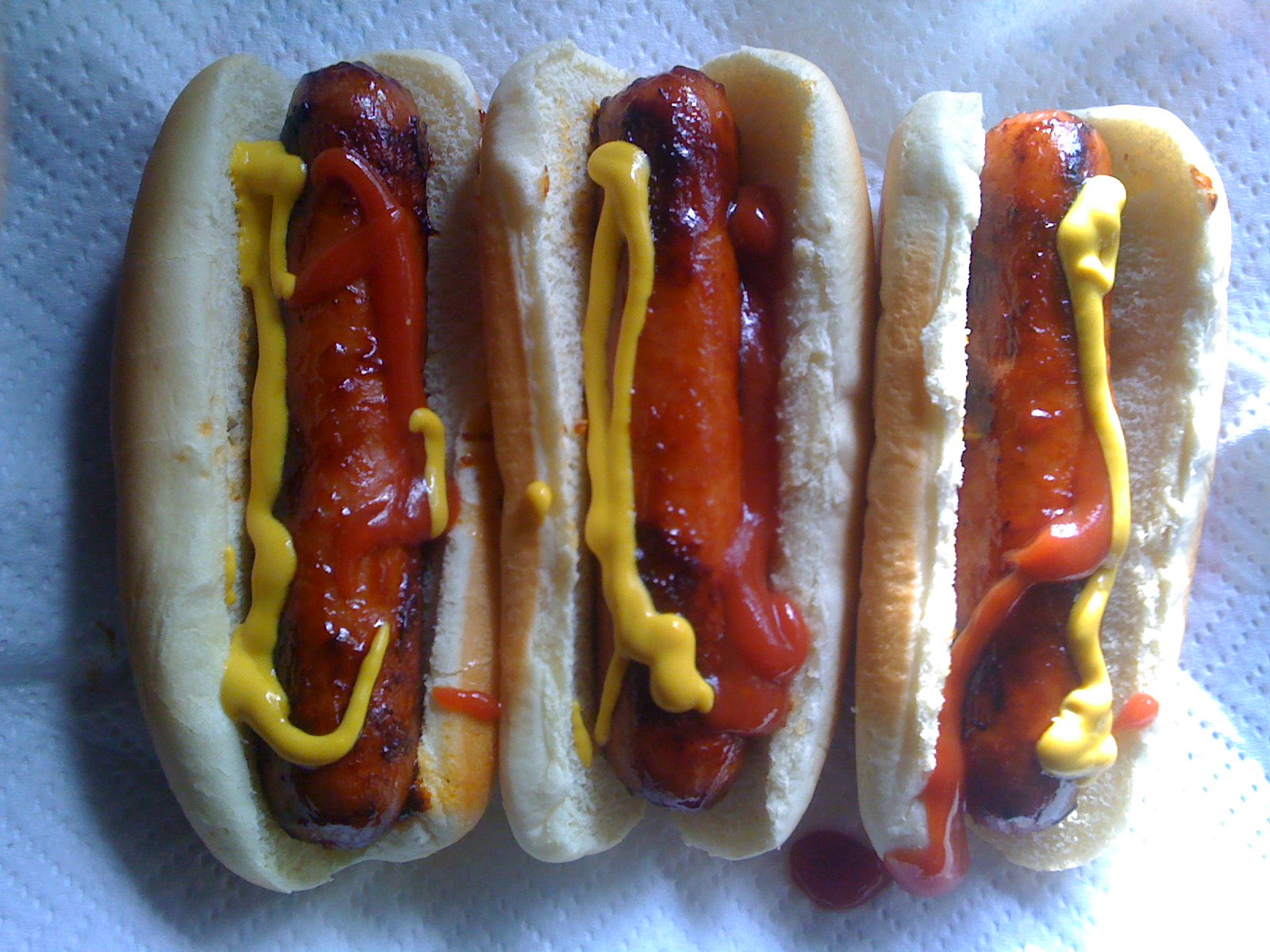This top-down photograph captures three grilled hot dogs nestled in toasted buns, each positioned vertically in the middle of the frame. The hot dogs exhibit characteristic char marks from the grill, enhancing their browned, slightly burnt appearance which evokes a tasty flavor expectation. Shiny with natural juices and topped with generous, somewhat haphazard stripes of ketchup and mustard, these hot dogs are visually inviting and ready to be eaten. The white bread buns, lightly toasted, cradle the juicy hot dogs. A slight spill of ketchup from the rightmost hot dog trickles onto the textured paper towel that serves as a simple background for the shot. The absence of any additional text or toppings such as onions or relish keeps the focus purely on the classic American snack, ready for an enjoyable meal.